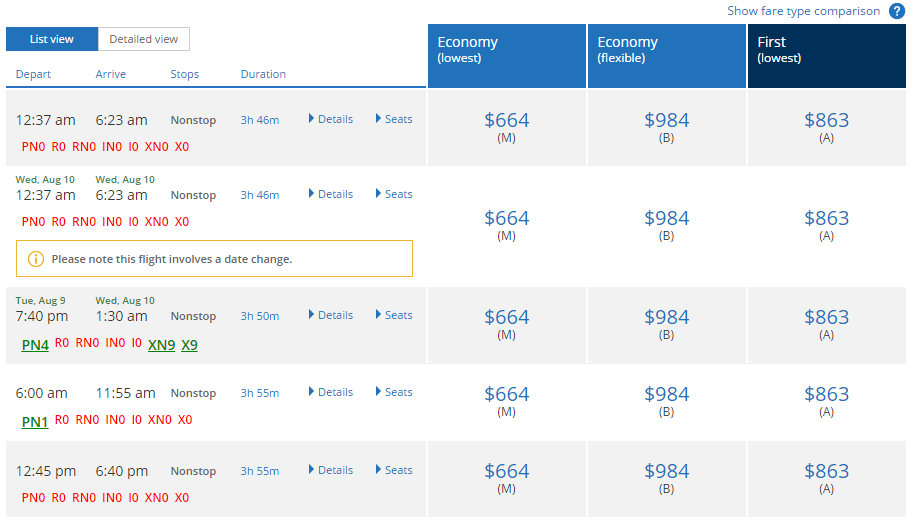In this image, we see a screenshot of a flight comparison interface. In the upper left-hand corner, there are two buttons: 'List View' on the left, which is currently selected, and 'Detail View' on the right. In the upper right-hand corner, there is a text prompt that reads "Show fare type comparison" accompanied by a question mark button to its right.

Dominating the left side of the screen is a large chart labeled with the following headers: 'Depart,' 'Arrive,' 'Stops,' and 'Duration.' Adjacent to these columns, on the right, are the labels 'Economy Lowest,' 'Economy Flexible,' and 'First Lowest.' The top row of the chart displays flight information: 12:37 a.m. departing, 6:23 a.m. arriving, non-stop, with a duration of 3 hours and 46 minutes. The corresponding prices for this flight are listed as $664 for Economy Lowest, $984 for Economy Flexible, and $863 for First Lowest.

All pricing options are consistent across every row, while the times of departure, arrival, and the duration vary under each listing on the left-hand side.